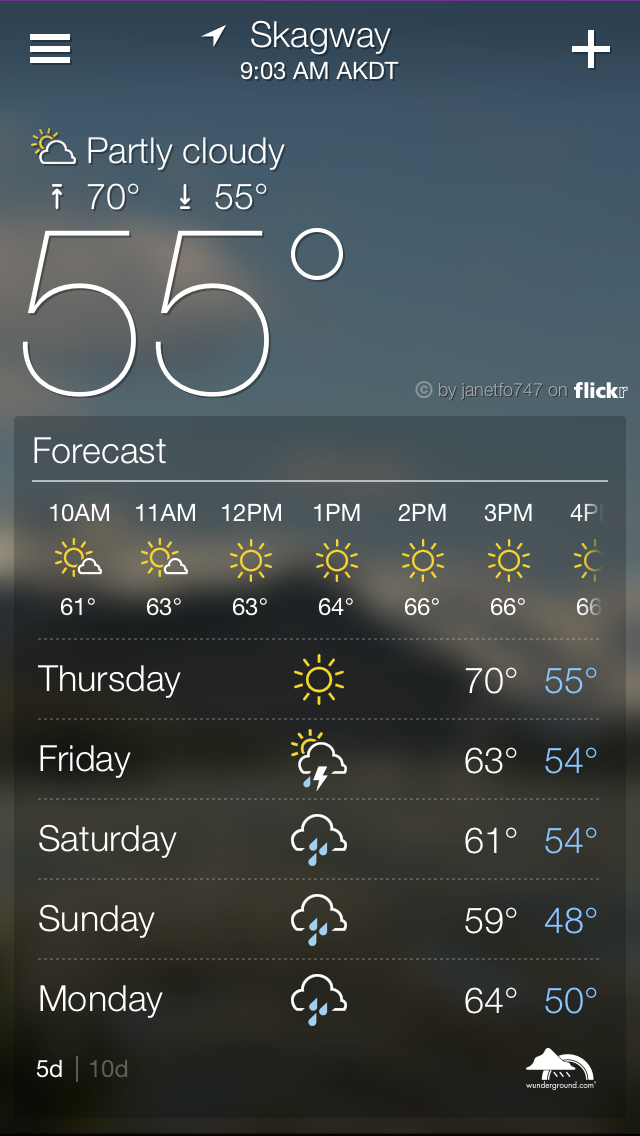This image is a detailed screenshot of a weather app displaying the current and upcoming weather forecast for Skagway at 9:03 AM. The current weather conditions indicate it is partly cloudy, with a temperature of 55 degrees Fahrenheit. The app's interface features a hamburger menu button located in the top left corner.

The hourly forecast for the day begins at 10 AM with a temperature of 61 degrees, rising to 63 degrees at 11 AM and maintaining 63 degrees at 12 PM. By 1 PM, the temperature increases slightly to 64 degrees, reaching 66 degrees at 2 PM, and staying consistent at 66 degrees through 3 PM and 4 PM.

Additionally, the 5-day forecast is provided: 
- **Thursday**: Sunny with a high of 70 degrees and a low of 55 degrees.
- **Friday**: A chance of thunderstorms with lightning, a high of 63 degrees, and a low of 54 degrees.
- **Saturday**: Rainy with a high of 61 degrees and a low of 54 degrees.
- **Sunday**: Rainy with a high of 59 degrees and a low of 48 degrees.
- **Monday**: Rainy again, with temperatures reaching a high of 64 degrees and a low of 50 degrees.

The app also has an option to switch to a 10-day forecast, located in the bottom right-hand corner of the screen.